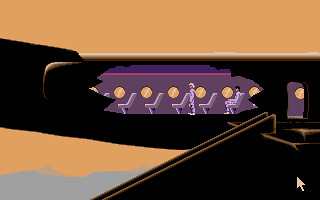A vibrant, cartoon-style illustration depicting a cross-section view of an airplane wing. The background features a warm, orangey-tan hue, accentuating the contrast with the black body of the airplane, which has a jagged, ripped-open section offering a peek inside the cabin. Within the exposed interior, the walls and seats are shaded in a muted purple-gray color. Bright orange circles adorn the walls, adding a whimsical touch. The cabin reveals two passengers: one seated and another standing, engaged in what appears to be quiet conversation. At one end of the plane, a small door is visible, leading to a dark, black area that transitions into a staircase descending towards a gray section of the image. The interplay of colors and the detailed elements evoke a sense of curiosity and unexpected adventure within the confines of this stylized aircraft illustration.